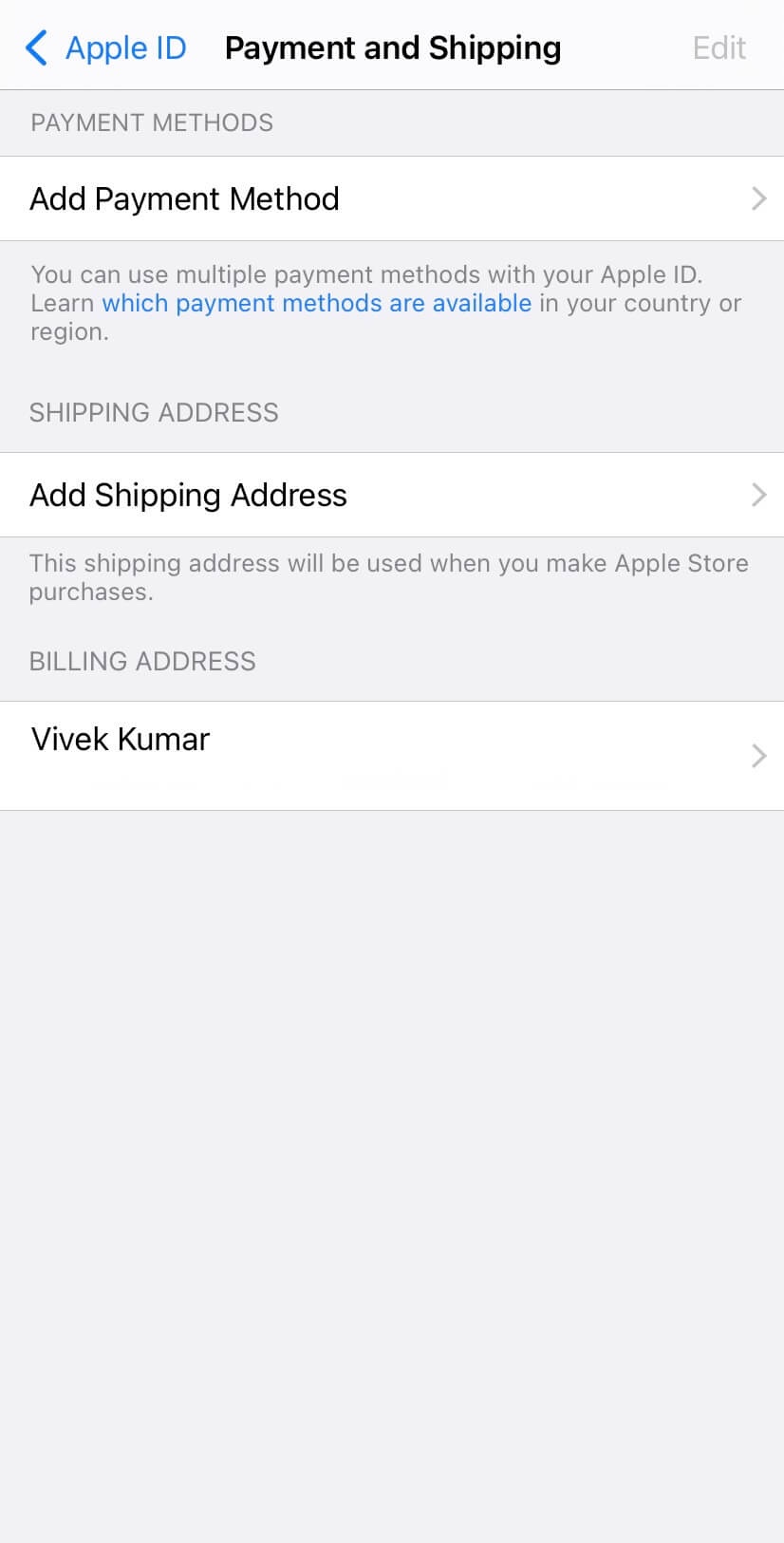The image depicts a screen, likely from a phone, displaying various settings related to Apple ID, payment methods, and shipping addresses. At the top, there is a header labeled "Apple ID, Payment, and Shipping" in black text on a white background. Below this header, the screen is organized into several sections with alternating background colors: white and very light gray. 

The first section titled "Payment Methods" is on a light gray background, followed by an option to "Add Payment Method" on a white background with a gray caret pointing to the right. Information about the availability of different payment methods by country or region is highlighted in blue text.

Next, there's a section for the "Shipping Address" on a light gray background, followed by an "Add Shipping Address" option on a white background, also accompanied by a gray caret to the right. This shipping address is intended for use with Apple Store purchases.

Further down, there's a "Billing Address" section, displaying what seems to be a name, "B-I-V-E-K-K-U-M-A-R," in black text on a white background, with yet another gray caret pointing to the right.

Much of the text is colored in either black, gray, or blue, depending on its function and importance, with important links or information such as "Apple ID" and "which payment methods are available" presented in blue.

Towards the bottom, the screen contains a large, almost square block of solid gray, which appears to be empty and devoid of content. The layout and presentation strongly suggest that this is a screenshot from a phone.